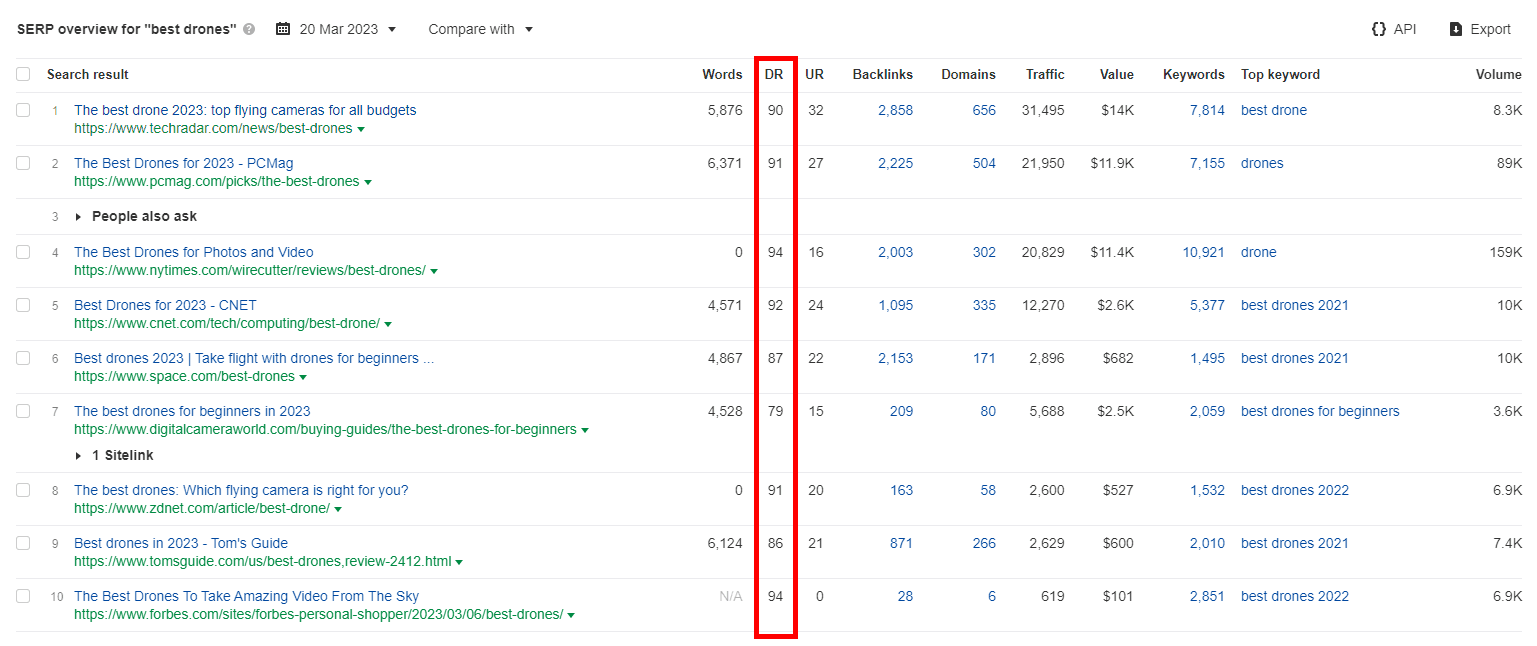**Image Description: SERP Overview for "Best Drones" Listings**

The image is a detailed screenshot of a search engine results page (SERP) overview for the query "best drones," captured on March 20th, 2023. The background is white, and the text is in black, with the content arranged in a tabular format showcasing ten search listings. 

Across the top, there are two dropdown menus: one indicating the date "March 20th, 2023," and another titled "Compare With." This section is labeled "SERP Overview for 'Best Drones.'"

Each listing in the table provides comprehensive information, including parameters such as Domain Rating (DR), URL Rating (UR), number of backlinks, referring domains, organic traffic, value of the listing, number of keywords, top keyword, and search volume. The list captures the following articles:

1. **The Best Drone 2023: Top Flying Cameras for All Budgets**
2. **The Best Drones for 2023** - PC Mag
3. **The Best Drones for Photos and Video**
4. **Best Drones for 2023** - CNET
5. **Best Drones 2023: Take Flight with Drones for Beginners**
6. **The Best Drones for Beginners in 2023**
7. **The Best Drones: Which Flying Camera is Right for You?**
8. **Best Drones in 2023** - Tom's Guide
9. **The Best Drones to Take Amazing Videos from the Sky**

This screenshot provides a helpful snapshot of the competitive landscape for articles reviewing the best drones, allowing for a quick comparison of key metrics for each listing.